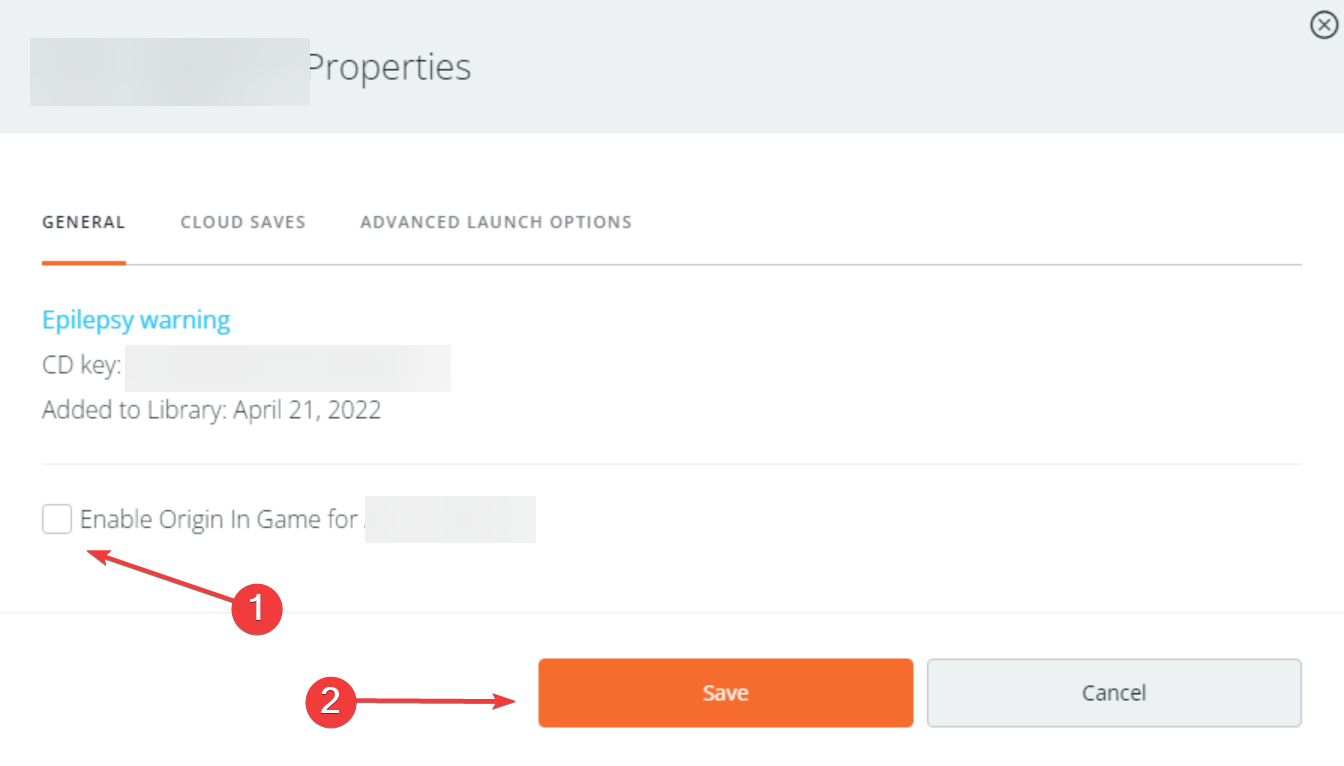At the top of the image, there is a large gray rectangle containing the word "Properties" in black letters, though the "P" is slightly obscured by a smaller overlapping gray rectangle. The right corner of the top section also features a black circle with a black "X" inside it.

Beneath the top banner, the left column lists several items vertically: "General," "Epilepsy Warning," "CD Key," "Add to Library April 21st, 2022," and "Enable Origin In Game 4." Adjacent to the "Enable Origin In Game 4" entry is a red circle with the number "1" inside it. An arrow extends from this circle, pointing towards a square box outlined in gray next to the "Enable Origin In Game 4" text.

To the right of the "General" heading, there are additional sections labeled "Cloud Saves" and "Advanced Launch Options" horizontally. Next to the "Enable Origin In Game 4" is a blank gray rectangle. Below it, there is another red circle labeled "2," with an arrow pointing right towards a red rectangle with the word "Save" in white letters. Adjacent to this red rectangle is another gray rectangle labeled "Cancel" in black letters.

A red portion of a horizontal gray line is located under the word "General" and stretches across the page, transitioning to gray beneath the "Cloud Saves" and "Advanced Launch Options" sections.